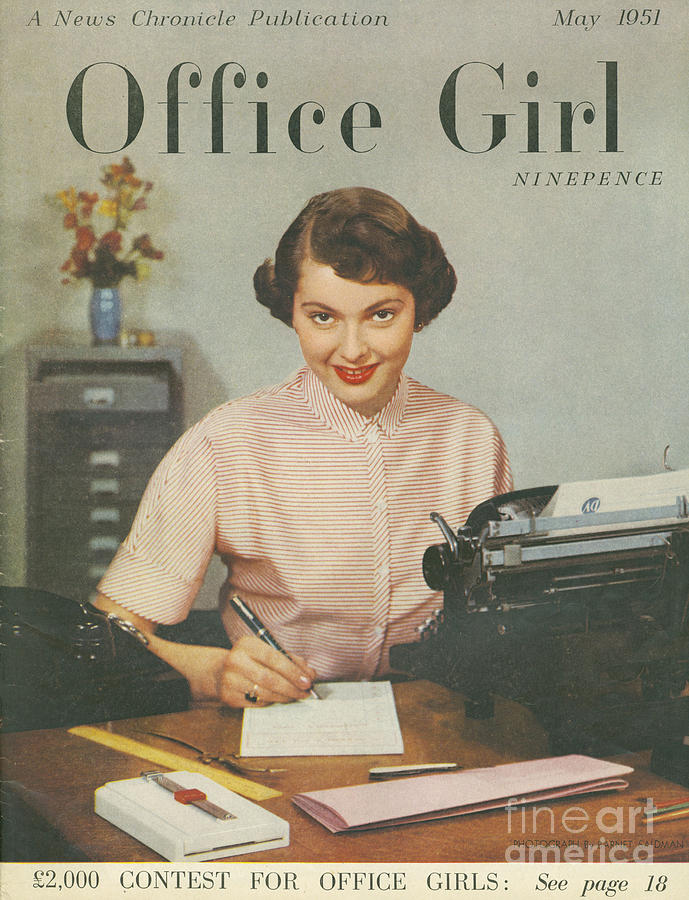The image depicts the cover of a magazine titled "Office Girl," a News Chronicle publication from May 1951, priced at ninepence. Central to the image is a woman with short brown hair, styled in a 1950s fashion, and adorned with red lipstick. She is seated at a desk, smiling directly at the camera. She wears a red and white striped collared button-up short-sleeve shirt. In front of her, she writes with a black pen on a white notepad. The desk features a black rotary phone on the left and a typewriter on the right, along with various other objects. The top of the page prominently features the magazine's title, "Office Girl," and a header for a 2,000 Pounds Contest for Office Girls, directing readers to see page 18.